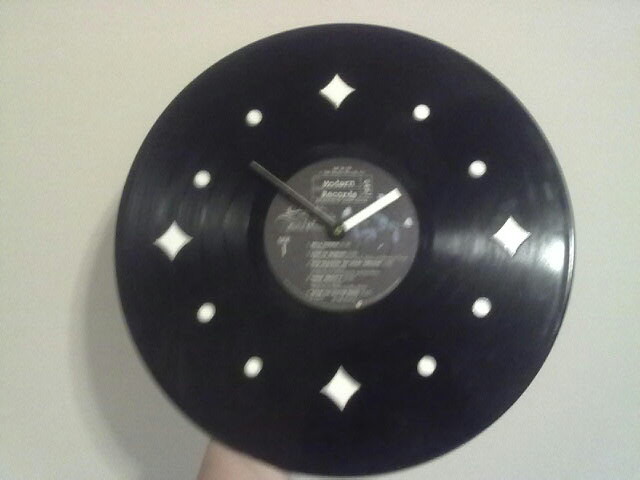The image features a unique clock crafted from a vintage LP record. The background is a gray wall, which is rectangular and unadorned, providing a neutral backdrop that emphasizes the clock's intricate details. A hand or arm is holding the clock up. The LP is circular, with visible ridges that catch the light, reminiscent of its intended use for playing music. In the center of the record, a label reads "Modern Records," although the song titles underneath are too blurry to discern. This clock does not have traditional numbers; instead, it uses white diamond markers at the 12, 3, 6, and 9 o'clock positions. The hours 1, 2, 4, 5, 7, 8, 10, and 11 are marked by small circles. The time displayed on the clock is approximately 1:53.